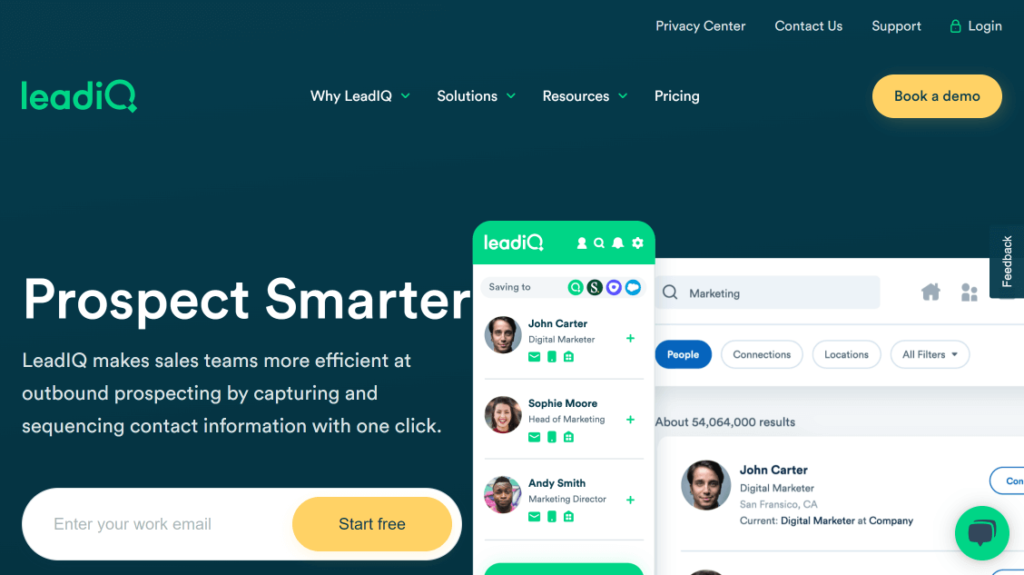The screenshot captures a detailed view of the LeadIQ web page, which prominently features a dark bluish-green background contrasted by the light green "LeadIQ" logo. The main navigation bar includes dropdown menus for "Why LeadIQ," "Solutions," and "Resources," alongside a direct link to "Pricing." Above this menu, starting from "Pricing" and moving right, the header contains links to the "Privacy Center," "Contact Us," "Support," and a "Login" button accompanied by a green lock icon.

Directly beneath the navigation bar is a prominent oval button labeled "Book a Demo" in blue text. The middle-botto left section of the page boasts a bold tagline, "Prospect Smarter," indicating that LeadIQ enhances the efficiency of sales teams in outbound prospecting and the seamless capture and sequencing of contact information with a single click.

Toward the bottom, there is a white input bubble prompting users to "Enter your work email," paired with a yellow "Start Free" button. An image of a mobile phone display features the LeadIQ app interface, highlighting contacts John Carter, Sophia Moore, and Andy Smith, with respective titles such as Digital Head of Marketing and Marketing Director. The app shows options to refine marketing searches by selecting people, connections, locations, and filters, with John Carter being actively listed.

Additionally, a chat button with a green outline and blue chat bubbles is situated in the bottom right corner, and a blue "Feedback" button with white text is positioned towards the upper middle right side of the screen, suggesting functionality aimed at assisting users in recruitment and job-related queries.